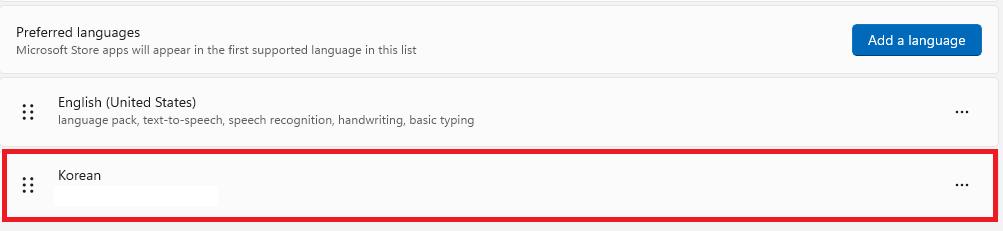This is a detailed horizontal screenshot with a white background and a gray outline at the top. The bottom section of the screenshot has a rectangular area outlined in red, also with a white background. 

At the top left, it displays the text "Preferred languages. Microsoft Store apps will appear in the first supported language in this list." On the top right, there is a blue rectangular button with white text in the center that reads "Add a language." Below this section, there are two columns of three vertical dots each. To the right of these dots, the text reads, "English (United States): Language pack, text-to-speech, speech recognition, handwriting, basic typing." 

On the far right of this line, there are three horizontal dots. Beneath the red-outlined section, another two columns of three vertical dots each can be found. To the right of this set of dots, it says "Korean." On the far right end of this line, another set of three horizontal dots is visible.